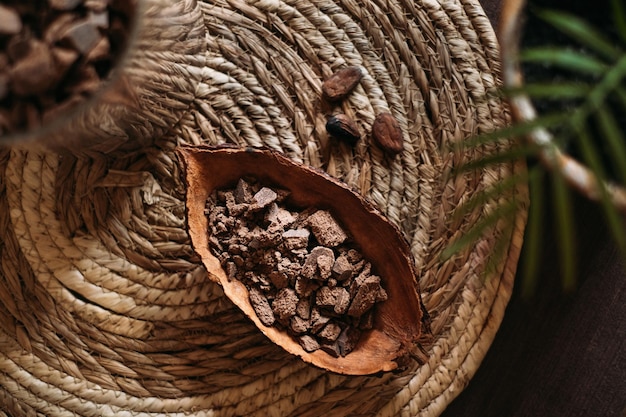In a dimly lit ambiance with a dark backdrop, a meticulously woven circular mat, crafted from tan and light brown roped material, serves as the focal point. Atop this mat rests an intricate half-open pod, resembling a large carved nut shell, filled with a collection of small grayish rocks, some broken, adding to its textured appearance. Adjacent to the pod lie three coffee bean-like seeds, enhancing the earthy color palette dominated by various shades of brown. In the upper left corner, a faint reflection hints at a glass object, while the top right corner showcases the blurred, green fronds of a fern-like potted plant with a white-rimmed pot, subtly encroaching into the scene.